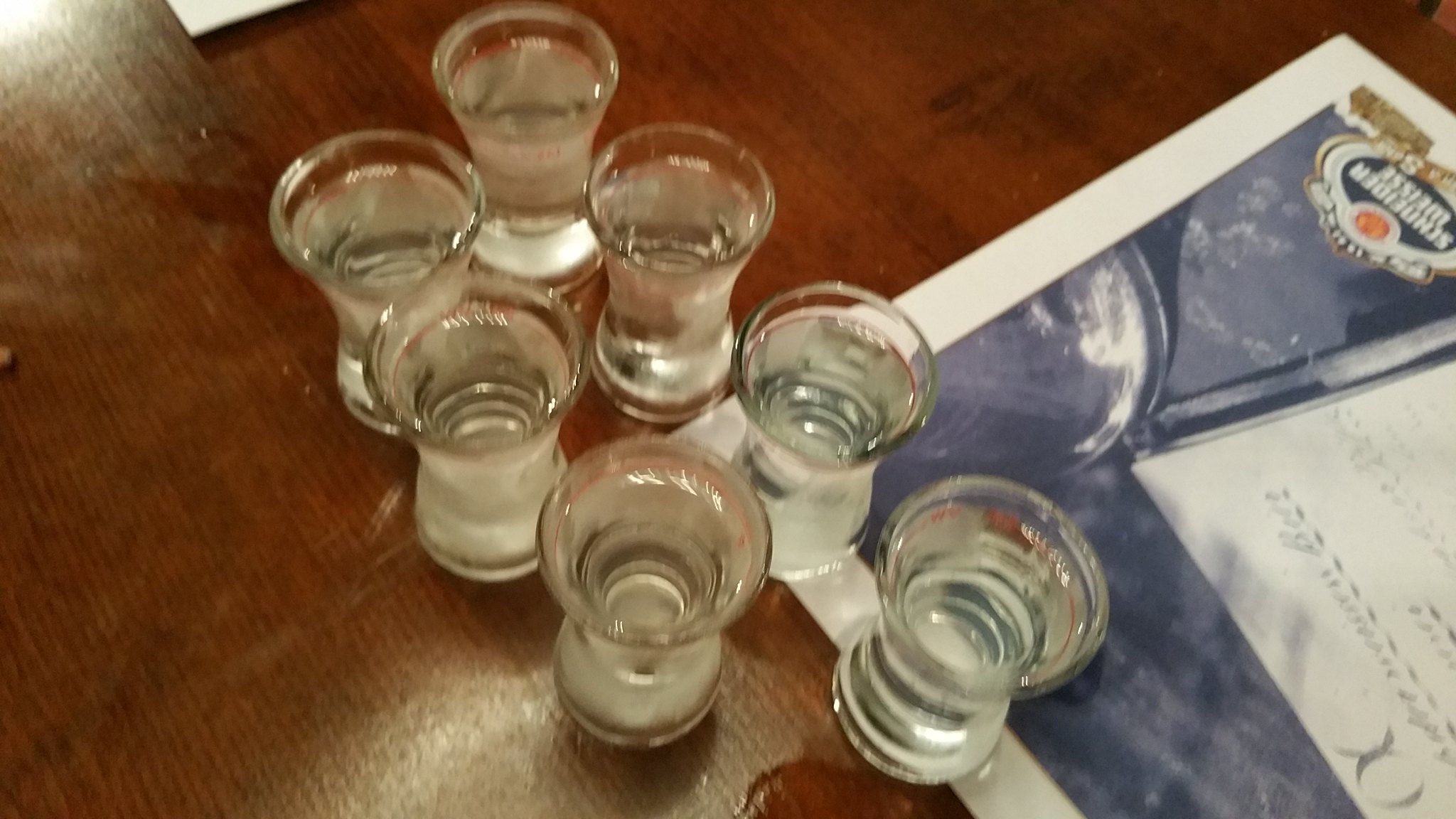The photograph captures a slightly out-of-focus arrangement of seven hourglass-shaped shot glasses, neatly lined up on a brown wooden tabletop. Each clear glass is filled to the brim with a transparent liquid, perhaps water or clear alcohol. A small wet spot is visible near one of the shot glasses at the bottom center of the image. The glasses are positioned in pairs, angled from the top left toward the bottom right of the photo. Some of these glasses overlap partially with a rectangular piece of paper on the left side of the image. This paper has a prominent white border framing an indistinguishable gray and blue image, adorned with an oval logo or seal in hues of white, orange, tan, and dark blue in the corner. The top left corner of another piece of paper also peeks into the frame. Light reflects off the glass and papers, adding subtle highlights to the scene, creating an overall casual yet intriguing visual narrative.